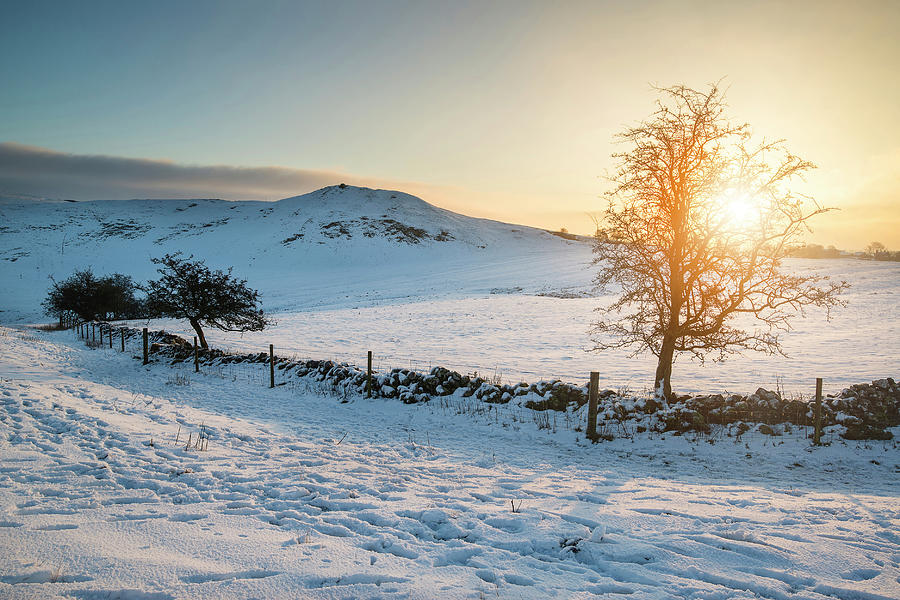The image captures a serene, snow-covered landscape devoid of people. The snow, untouched in most areas, is punctuated by tracks—perhaps from some vehicle—creating a series of lines and holes. Various twigs peek through the blanket of white, adding texture to the scene. A rustic wooden fence with posts connected by horizontal lines stretches into the distance on the left, gradually fading into the horizon. Beyond this fence, a cluster of trees and bushes is visible. On the right side, a larger, seemingly lifeless tree stands starkly against the brilliantly shining sun, positioned in the sky. A mixture of yellow and blue hues colors the sky, likely indicating early morning or late afternoon, with the blue intensifying towards the upper left corner. Ominous dark clouds loom in the sky above a higher hill area on the left, adding a dramatic contrast to the otherwise tranquil winter scene.